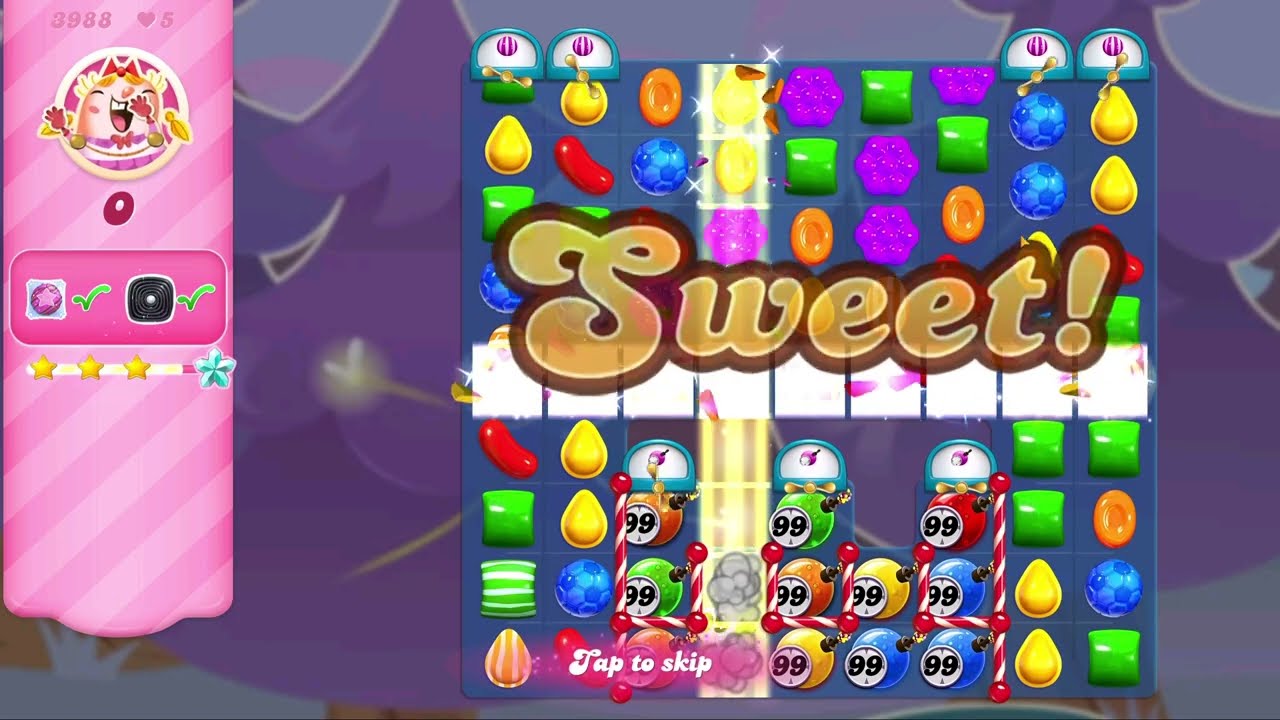Here is a detailed caption combining and refining the given descriptions:

---

The screenshot captures a vibrant, colorful moment from a mobile game reminiscent of Candy Crush. Dominating the right side of the horizontal image is a large, square grid divided into approximately 10 columns, each filled with various colorful objects that resemble fruits and candies. Among these objects, specific items such as lemon drops, purple flowers, green squares, blue soccer balls, green striped square candies, red tamale candies, and orange and white striped gumdrops are discernible. Central to the scene is a gold, semi-transparent text with a brown border, reading "sweet!" with an exclamation mark. This text overlays a highlighted fourth column from the left, indicating a scoring move.

On the left side of the screen, a pink rectangular banner with vertical striping features a circular profile image of a laughing cartoon character or creature. Above this character, there's text displaying the number 3988 with a heart symbol and a "5" next to it. Below, additional elements include two squares with green checkmarks—one containing a star, the other a speaker icon—and a row of three stars beneath them. The image suggests that a sequence or row has possibly been matched, leading to the elimination of colors or shapes, and the generation of special items to boost the player's score.

---

This caption integrates the repeated details from each speaker, providing a cohesive and comprehensive description of the captured game moment.